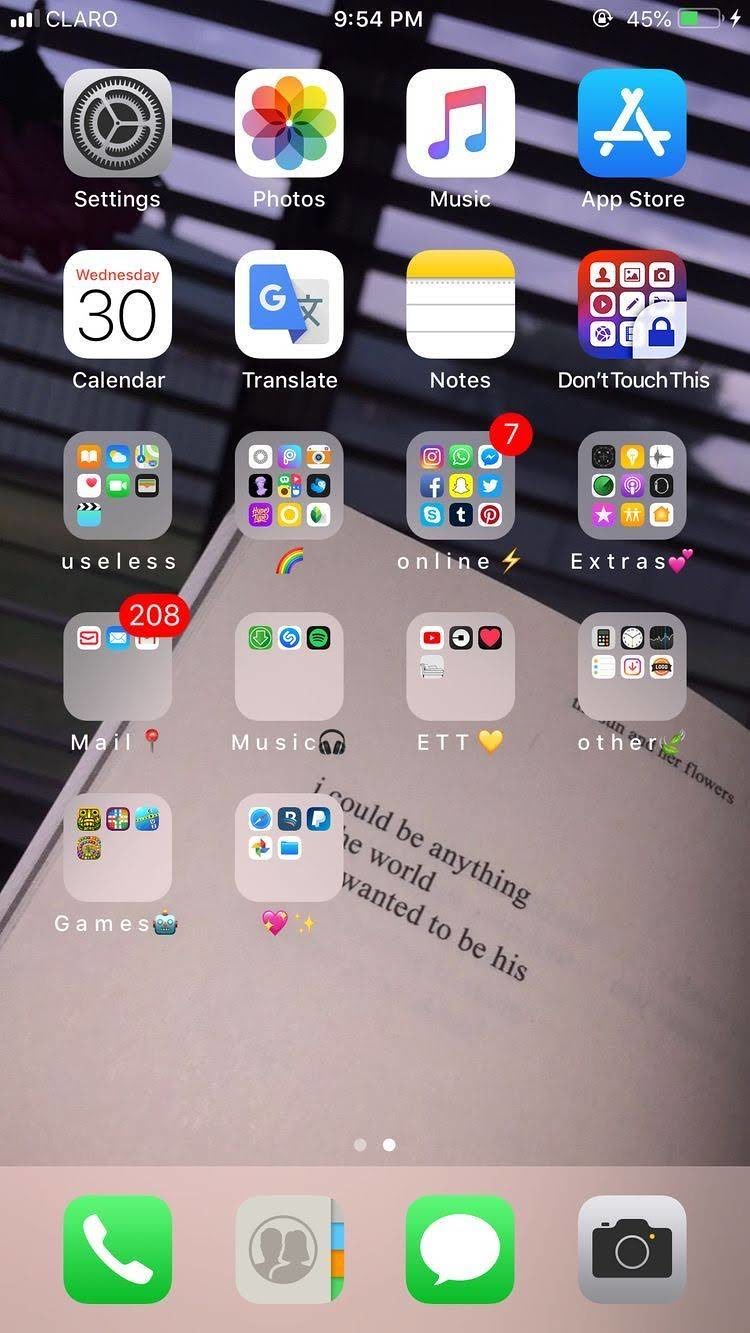This image is a screenshot of an iPhone home screen. The wallpaper shows a close-up of a partially open book, revealing a portion of a page with the text: "I could be anything. The world... wanted to be his." This text is partly obscured by app icons. 

At the top of the screen, the status bar indicates the phone is connected to the Claro network with three out of four signal bars filled. The current time is 9:54 p.m., and a lock icon shows that the phone is locked. The battery icon, displaying 45% with a lightning bolt, signifies that the phone is charging.

The home screen is organized into several rows of app icons and folders. The top row includes Settings, Photos, Music, and the App Store. The second row features Calendar, Translate, Notes, and a folder labeled "Don't touch this." 

Further rows contain additional folders and apps:
- A folder labeled "Useless"
- A folder with a rainbow label
- A folder labeled "Online"
- A folder labeled "Extras"
- A folder labeled "Mail"
- A folder labeled "Music"
- A folder labeled "ETT"
- A folder labeled "Other"

The bottom row contains two folders:
- One labeled "Games"
- One labeled with a heart and a star emoji

Each folder contains several apps, represented by their initial icons visible on the folders.